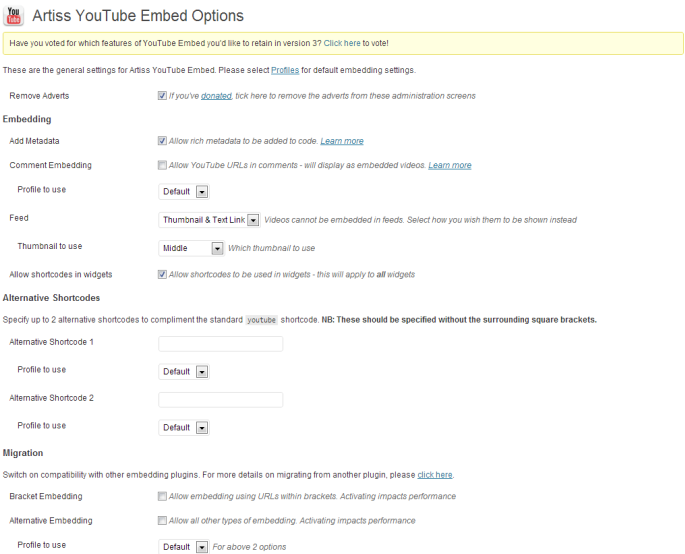The image displays the interface for Artist YouTube Embedded Options. In the upper left-hand corner, there's a label indicating "Artist YouTube Embedded Options." Just below the label is the YouTube logo, with 'You' in black font, 'Tube' in white font, and a red play button icon.

Directly beneath this, a bright yellow bar stretches across the width of the screen, prompting users with the message: "Have you voted for which features of YouTube Embedded you'd like to retain in version 3? Click here to vote."

Below the yellow bar, the text introduces the general settings for Artist YouTube Embedded, instructing users to select profiles for default embedding settings. The first section addressed is "Embedding," where there is an option "Add materials" which is checked off, indicating that rich metadata is allowed to be added to the code.

The subsequent section is titled "Alternative Shortcuts," and the final section is labeled "Migration." The layout and settings are clearly organized to assist users in configuring their embedded YouTube options efficiently.